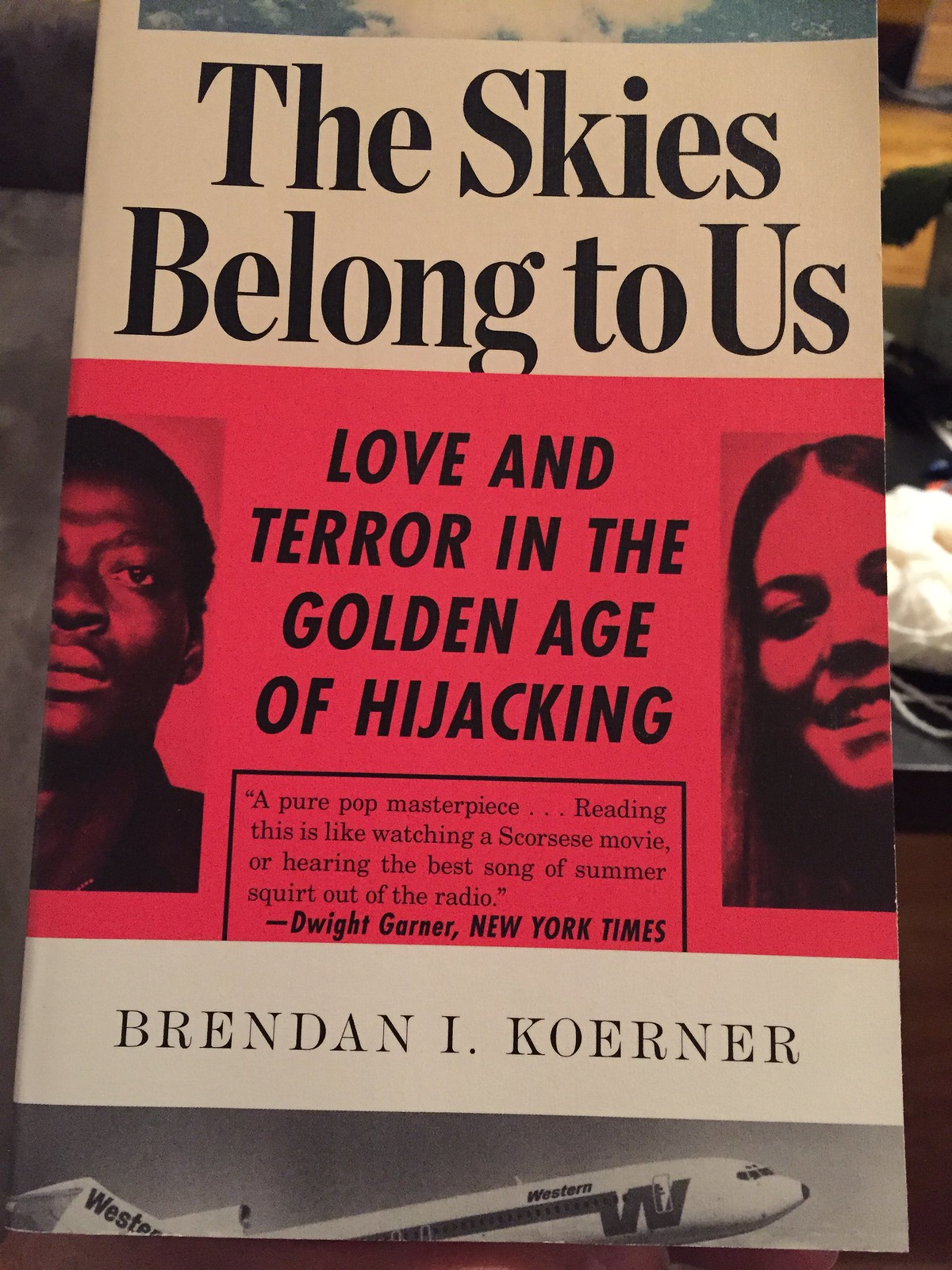The image appears to be a book or magazine cover with a striking design divided into distinct sections featuring varied colors and text. At the top, against a light brown background with black text, it declares, “The skies belong to us.” Below this, the central portion of the cover has a vivid red background with two figures: a Black man on the left, staring straight ahead, and a young Caucasian woman on the right, slightly tilting her head to the left, both flanking bold black text that reads, “Love and Terror in the Golden Age of Hijacking.” Beneath this section, there’s a black square containing a review, stating, “A pure pop masterpiece… this is like watching a Scorsese movie or hearing the best song of summer squirt out of the radio,” credited to Dwight Garner from the New York Times. Following this, text against a light gray background names the author, Brendan I. Koerner. At the bottom of the cover, a black and white image of an airplane with a white fuselage and the word “Western” emblazoned on it, along with a distinctive line ending in a ‘W’, further emphasizes the book’s aviation theme. The overall composition suggests a dramatic and visually arresting design suitable for a compelling narrative about a gripping and turbulent era.